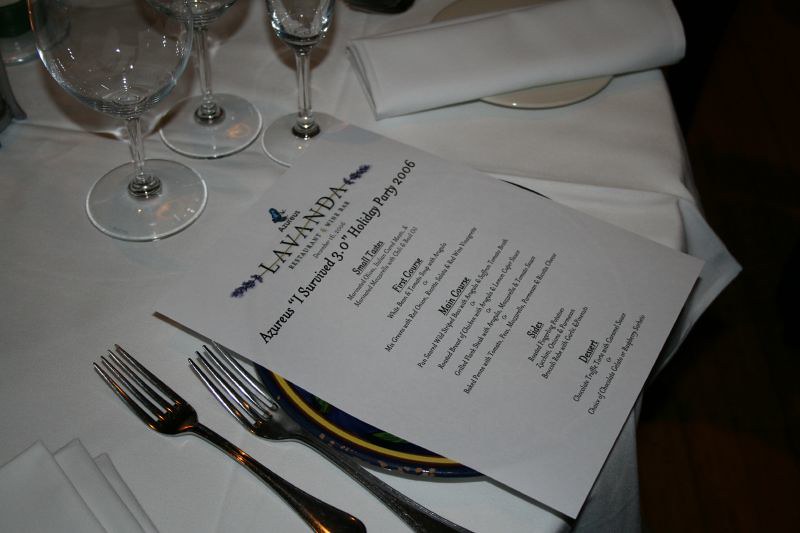In this elegant landscape image, a meticulously arranged dinner table is showcased, adorned with a crisp white linen tablecloth. Central to the composition is a place setting angled at 45 degrees, with the bottom closest to the bottom right of the image. This setting consists of two forks placed to the left of a pristine white plate, upon which lies a neatly folded menu. The menu, printed in classic black ink on white paper, details the offerings for "La Banda's Heart Holiday Party 2006" with the whimsical tagline, "I Survived 3.0." The courses are organized into "Small Tastes," "First Course," "Main Course," "Sides," and "Dessert."

Scattered across the table are several napkins: one distinctly visible in the bottom left corner and another from an adjacent place setting peeking from the top right. At the top left of the frame, three wine glasses are strategically arranged in ascending order of size—a large, a medium, and a small glass—awaiting to complement the meal's offerings. This scene exudes a sense of anticipation and festive sophistication, capturing the essence of a memorable culinary celebration.